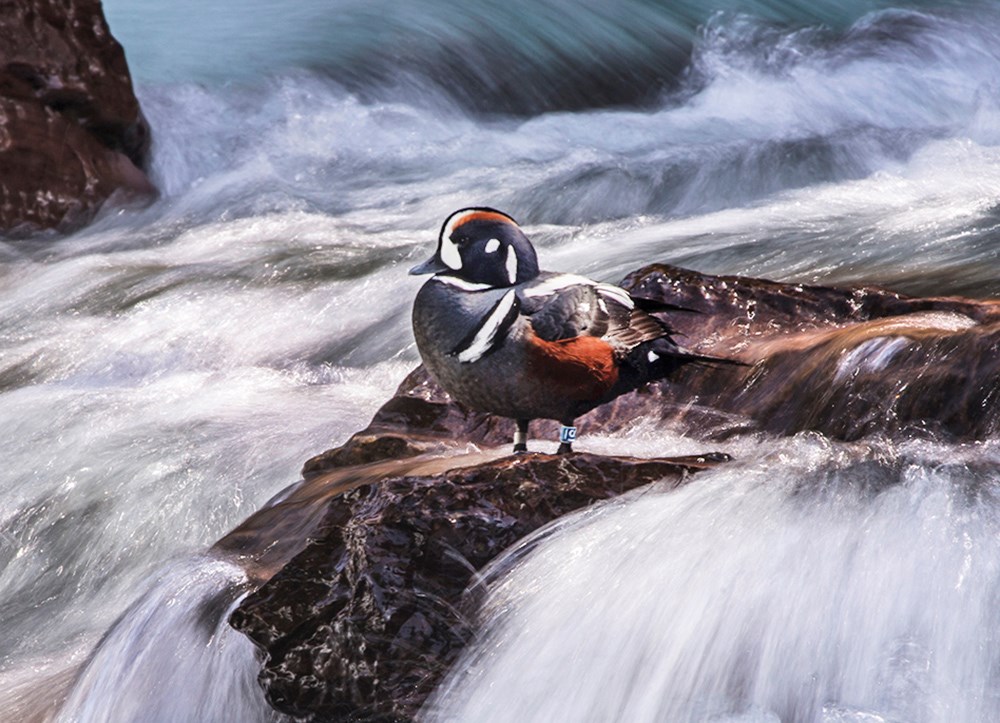This detailed illustration depicts a rapid, fast-moving stream with turquoise and gray swirling waters, dotted with white caps. The rough water cascades around several brown rocks with white demarcations, creating a dynamic scene filled with motion streaks indicative of the stream's speed. Perched on one of these central rocks, a small, rotund bird commands attention. It faces left, showcasing its striking plumage. The bird has a predominantly brown body with highlighted areas featuring red on its head and sides near its left wing, and white accents around its eyes, nose, and parts of its upper body. This vivid depiction, despite being an illustration rather than a photograph, captures a lifelike moment of this ornately colored bird amidst the untamed natural beauty of the rushing stream.